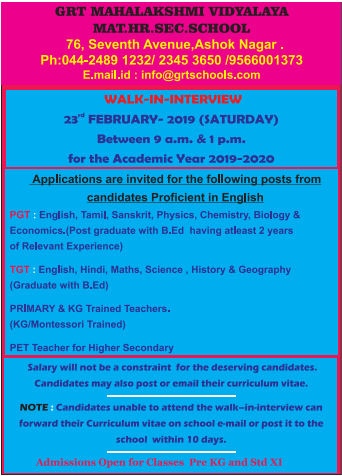The image is an informational poster with a visually striking red and pink theme, divided into two main sections. The upper section is predominantly pink, while the bottom section is blue. At the top of the poster, black text on the pink background reads, "GRT Mahalakshmi Vidyalaya Mathasek School." Below that, in yellow text, the poster provides the address: "76, 7th Avenue, Ashok Nagar."

In the blue section of the poster, the words "Walk-in Interview" are prominently displayed in red text. Additional details are provided in black text: "23rd February, 2019, Saturday between 9 a.m. and 1 p.m. for the academic year 2019 to 2020." The text further specifies, underlined for emphasis, that "Applications are invited for the following posts from candidates proficient in English."